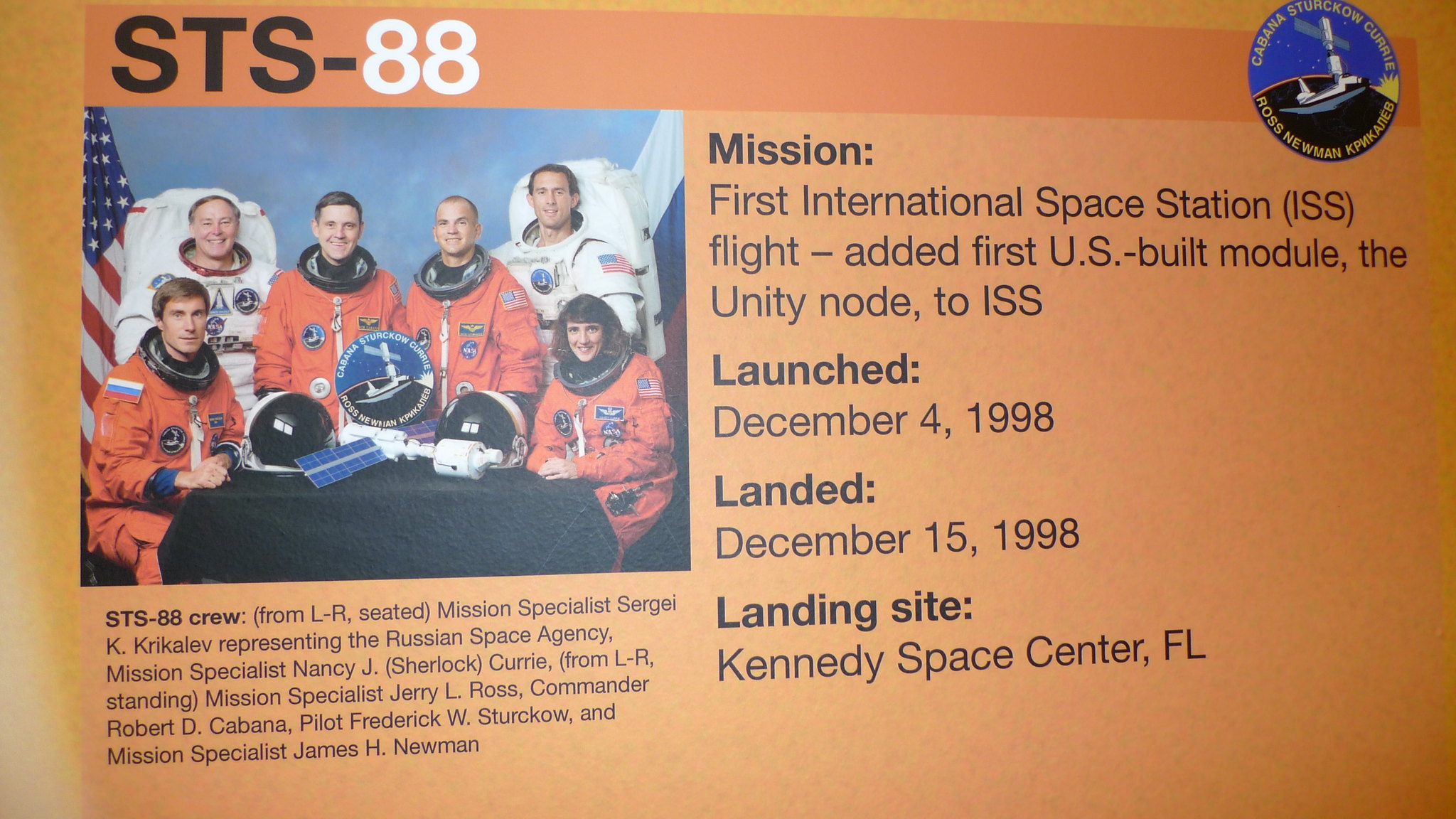This is a full-color print poster with a predominantly burnt orange background featuring a detailed depiction of the STS-88 mission. On the left side of the poster, there is a photograph of six astronauts—four in orange jumpsuits and two in white environmental suits. Among them are one woman and five men. The top of the image is marked by the headline "STS-88," with the subheading "STS-88 Crew," listing all crew members. To the left corner, there is an American flag, and in the right corner, another flag colored white, blue, and red, possibly representing another nation involved in the mission. In the center of the poster, a digitally edited logo featuring the Space Shuttle and the International Space Station (ISS) is displayed, although the surrounding text is hard to decipher. On the right side of the poster, there is mission information: "First International Space Station flight, added first U.S.-built module, the Unity node to ISS," with key dates—launched December 4, 1998, and landed December 15, 1998, at Kennedy Space Center, Florida. The overall look and arrangement of text and images suggest that this poster could be an informative display in a museum, delineating the historic significance of the STS-88 mission.